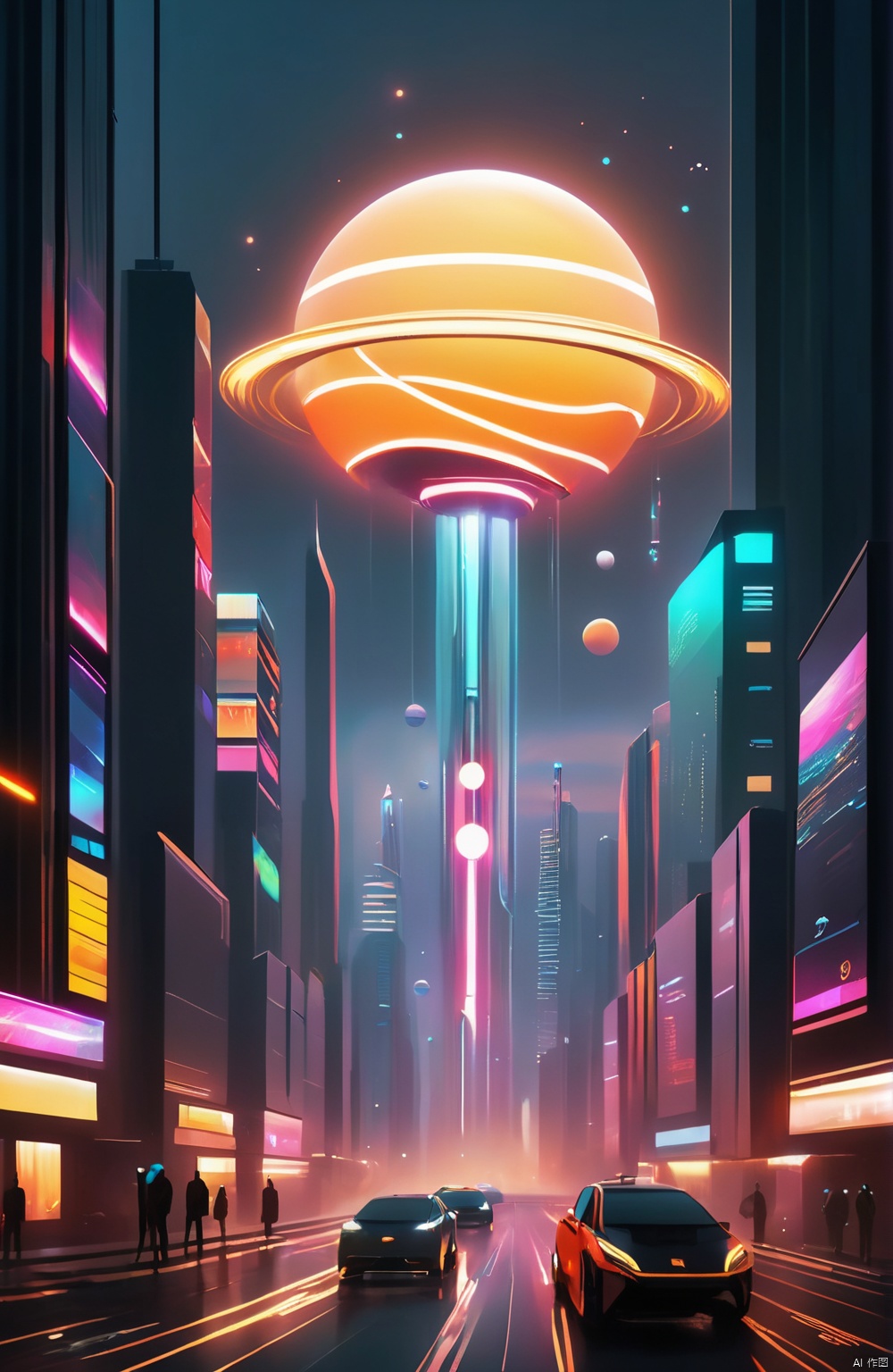The digital artwork portrays a vibrant, futuristic city street bustling with activity. In the foreground, sleek black cars with white headlights glide along a shiny black street, accentuated by glowing red strips. On either side of the street are black sidewalks, where shadowy pedestrians stroll. Tall, smooth buildings line both sides, adorned with illuminating panels in various colors including pink, yellow, and blue. 

In the distance, a striking blue-lit pole ascends to an orange sphere with distinctive white stripes, surrounded by an orange ring reminiscent of Saturn. The sphere, with its surreal presence, evokes thoughts of it descending like the New Year’s Eve ball in Times Square. Above, a dark gray sky adorned with twinkling white stars and additional floating orbs—orange, purple, and gray—add to the cosmic ambiance. Below, the street scene is alive with vivid hues of pink, yellow, blue, and gray, creating a colorful, game-like atmosphere suggestive of a digital rendering.